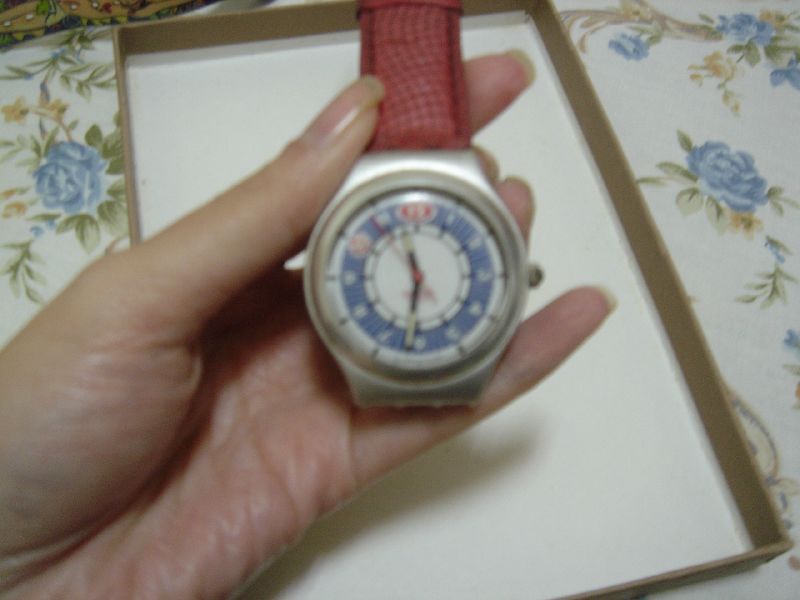An older, out-of-focus photograph captures a hand holding a silver, round watch with a distinctive face. The watch sports a braided red faux leather strap, which adds a touch of vintage charm. The watch face is blue with subtle stripes and features white numbers, with a red circle emphasizing the number 12. The person's hand, noticeably pale with unusually long nails, delicately holds the timepiece above a box lid resting on a table. The table is adorned with a tablecloth decorated with blue roses and green leaves, adding a floral background to the scene.